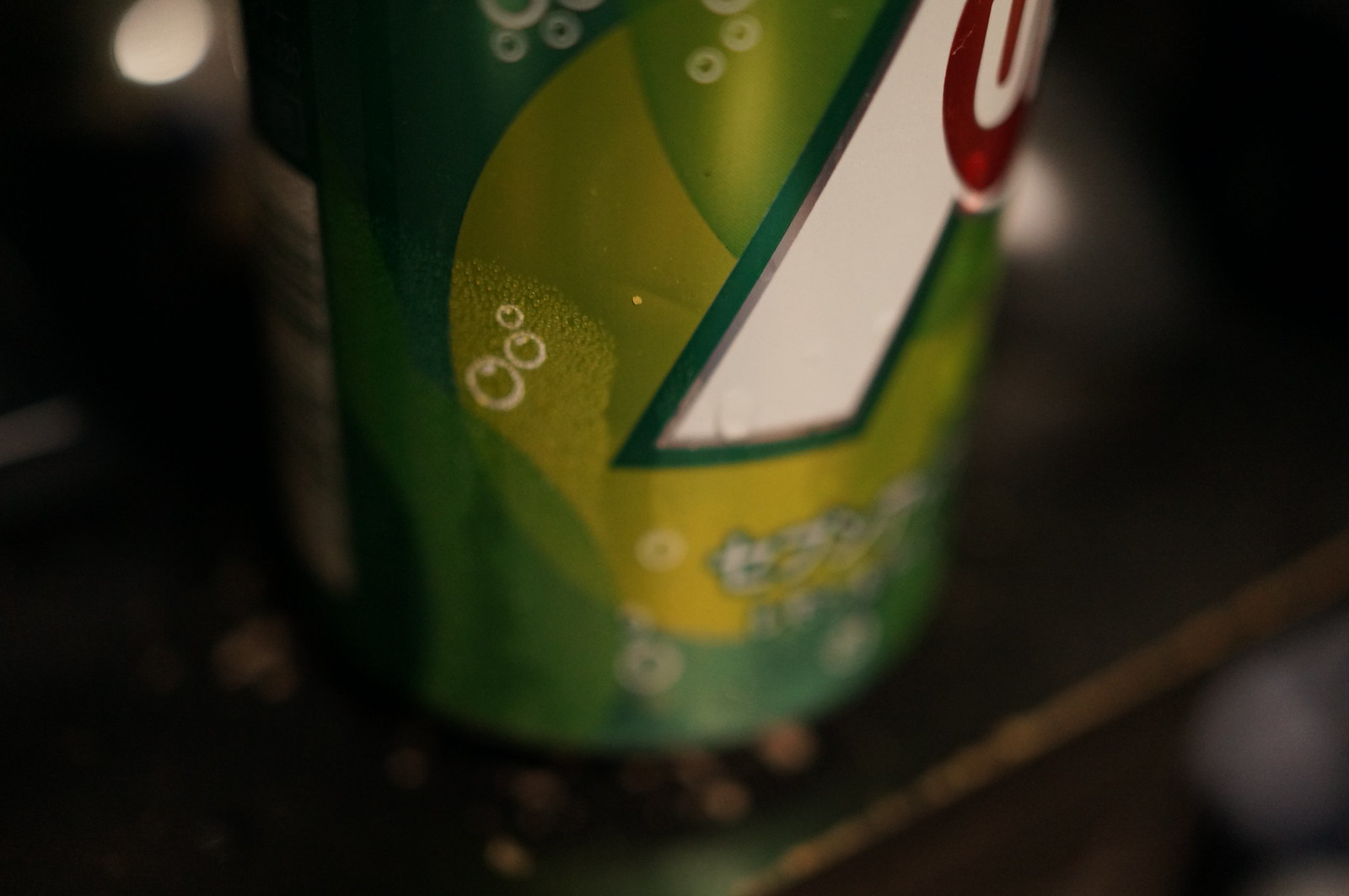The image depicts a close-up of a dark green aluminum can of 7-Up situated on what seems to be a dark wooden table with noticeable blemishes. The can features the recognizable 7-Up design elements: a partial view of the bottom portion of the white "7", as well as a segment of the red circle containing the white "U". The green hue of the can is interspersed with images of yellow and white bubbles. The lighting in the room appears dim, contributing to a generally dark appearance in the photograph. Despite the lack of moisture on the can suggesting it hasn't been refrigerated recently, it remains the central focus of the image. The background is heavily blurred, revealing only indistinct dark gray shadows and blacks with faint reflections of light in the upper left and bottom right corners.